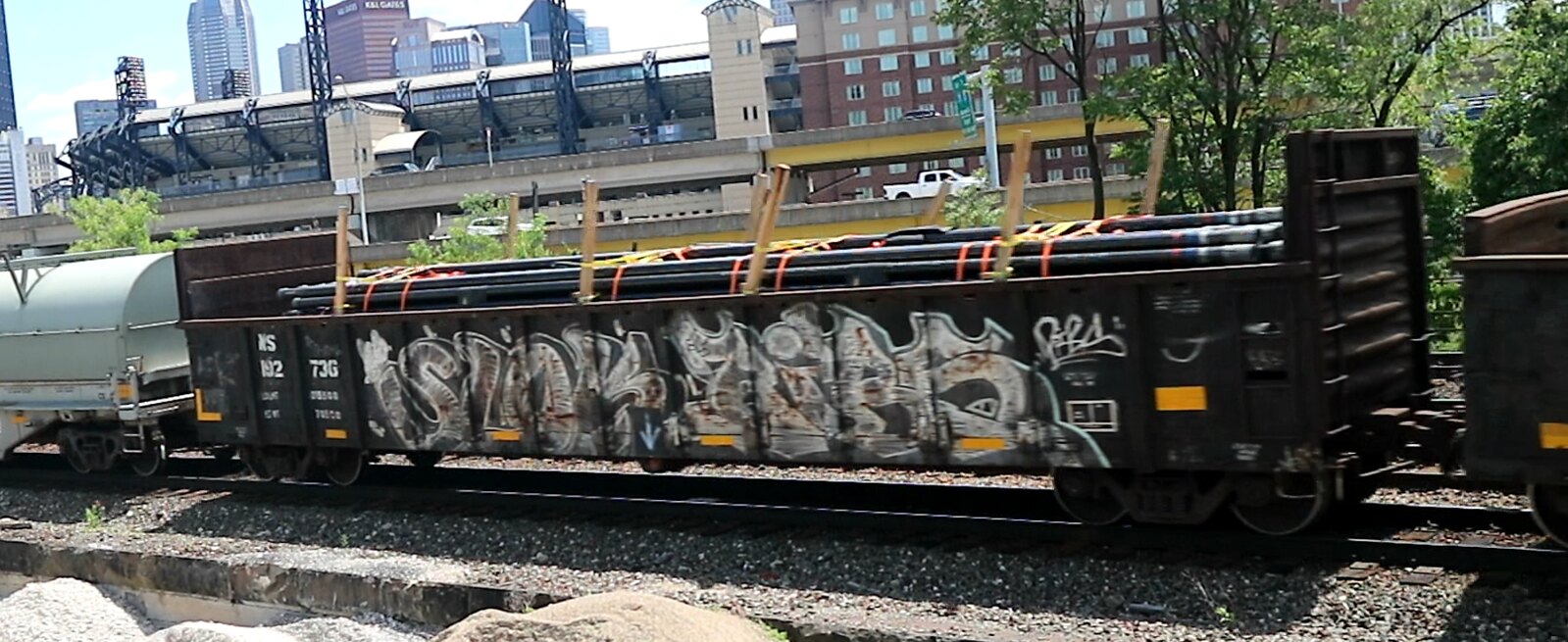The photo features a train with a black, open car prominently displayed, loaded with long black pipes secured by red or orange straps. The side of this train car is covered in large, white and yellow graffiti, with "SLOB" clearly visible and some indistinguishable numbers and letters, including "73G". A sequence of connected cars is seen, with a brownish and white container car designed for carrying liquids visible in the lineup. The train runs along tracks bordered by gravel and sand, with greenery and small trees to the right. In the background, there's a bustling cityscape featuring numerous high-rise buildings, including what appears to be an apartment building and a tunnel-like structure. Additionally, a white pickup truck is seen driving on an adjacent roadway.